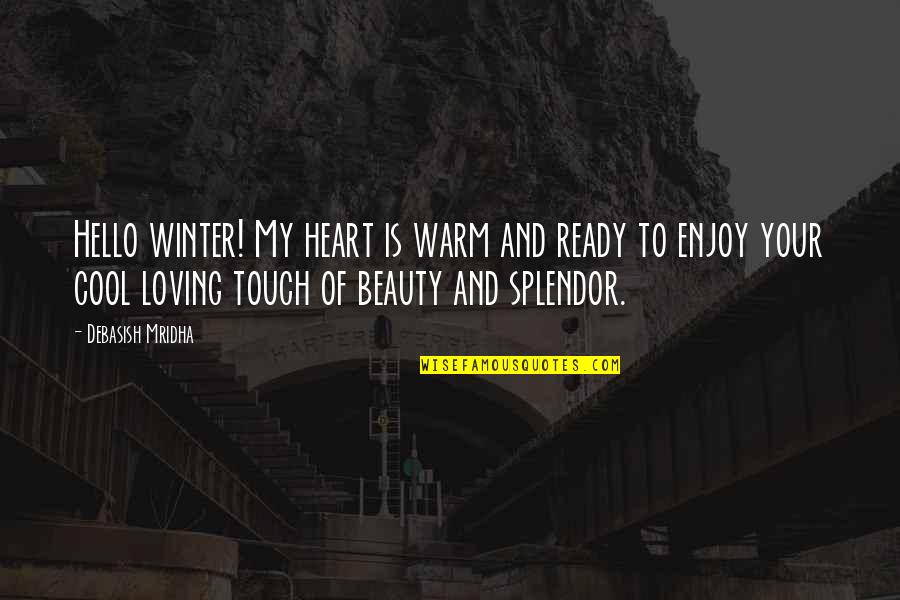The image captures a mysterious, somewhat industrial setting featuring a tunnel named "Harpier Ferry," built into the side of a rocky mountain. Two roofed, metallic paths or bridges extend from this tunnel towards the viewer. Above the tunnel, the rugged mountain rises majestically, adding to the dramatic atmosphere. Superimposed on the image in bold, white capital letters is an inspirational quote: "HELLO WINTER! My heart is warm and ready to enjoy your cool loving touch of beauty and splendor." The quote is attributed to Debasish Mridha, with his name also in white text, following a hyphen. Toward the right and near the middle of the image, there is a yellow rectangular bar with gray text that reads "wisefamousquotes.com." The quote and website details stand out sharply against the darker, moody backdrop, combining to deliver a message of warmth and appreciation for winter's beauty amidst an industrial landscape.